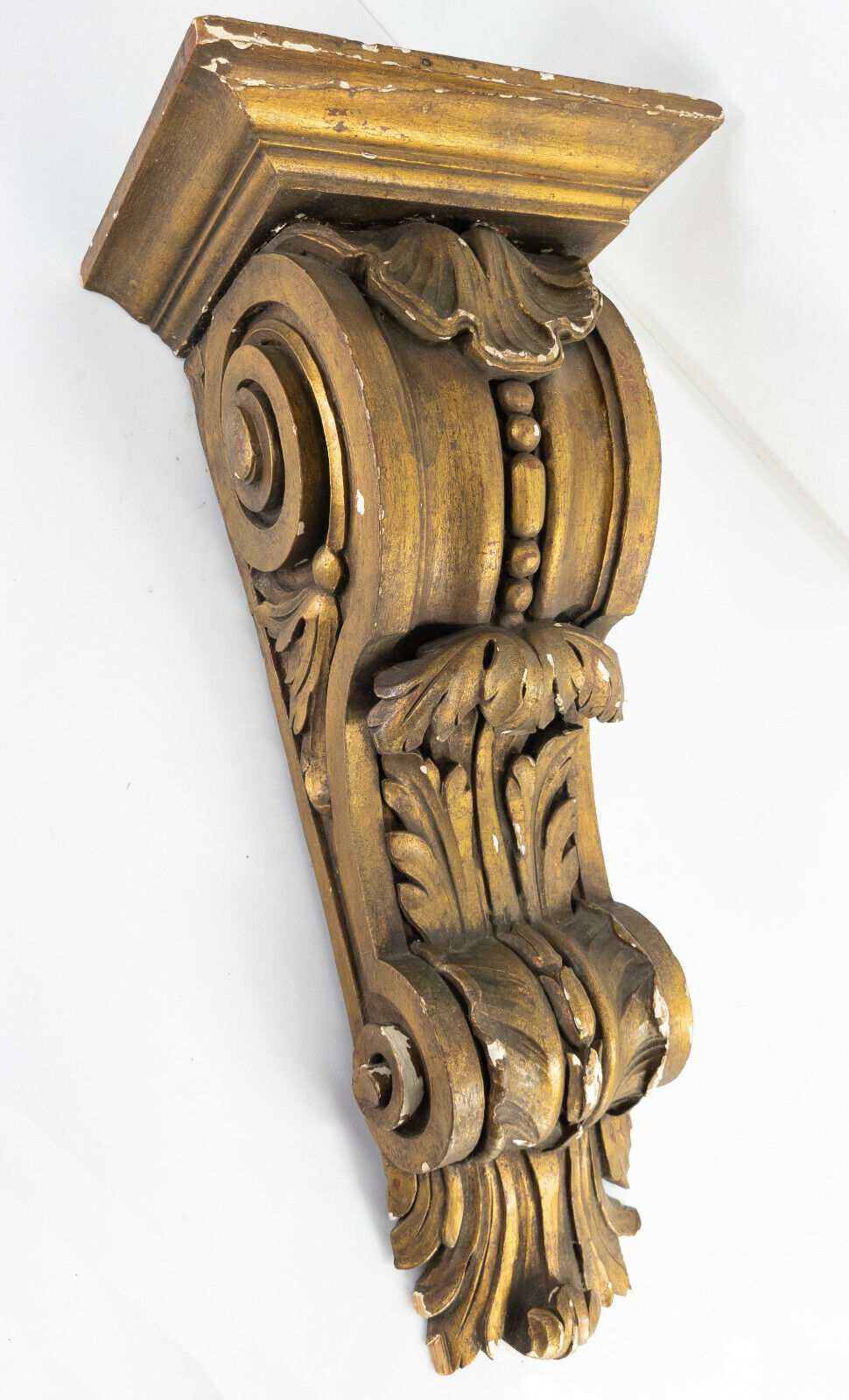This image captures an intricately carved wooden wall shelf with a distinctive 19th-century style. The shelf, likely made from medium blonde wood, serves as a decorative piece that is both functional and ornate. The structure features a short, square base on top, ideal for placing a vase or other small items. From this base, a long, vertically extended scrollwork descends, embellished with detailed carvings of leaves and circular designs. The central motif includes a pattern of beads—two small beads followed by one large bead and then repeating. This elaborate piece, which appears heavy and measures around two feet in length, is designed to be mounted on a wall and would complement spaces such as near a fireplace or under an awning. The background is a white wall with an angled ceiling that almost intersects with the shelf, emphasizing its prominence and historical charm.